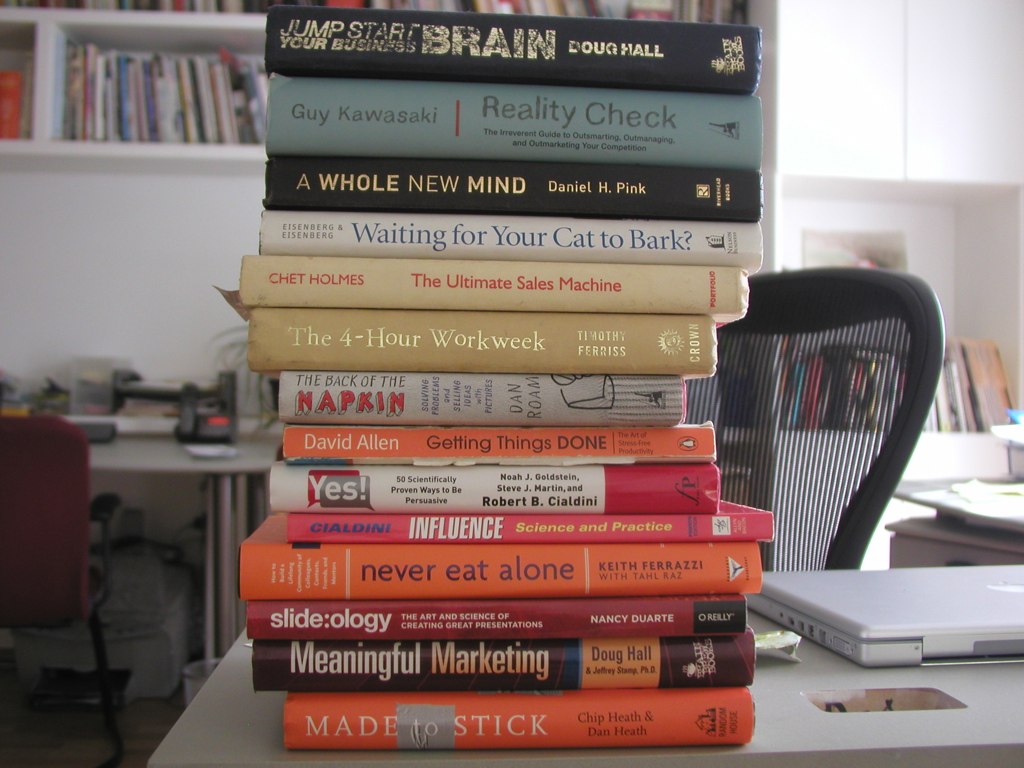The image portrays a large square scene set in a room that could either be a house or an office. Centrally, a stack of approximately 12 to 14 books is piled atop a light gray desk. The books are arrayed in an assortment of colors including orange, red, black, white, and several other hues. Notable titles in the stack include "Made to Stick" at the bottom in orange, followed by "Meaningful Marketing" in black, and titles like "Waiting for Your Cat to Bark," "The 4-Hour Workweek," and "The Ultimate Sales Machine," suggesting a mixture of marketing and sales themes.

To the right of the books, a closed silver Apple laptop is positioned, identifiable by the distinct Apple logo. Behind the desk, a black vented chair is partially visible. Moving to the background on the left side, another gray desk can be seen supporting a red cushion chair and a printer. Above this secondary desk, two bookshelves line the wall, filled with rows of neatly arranged books. The right side of the room features a white wall with a cutout area, where additional books are stacked vertically. The setting is undeniably indoors, exuding the atmosphere of a detailed and organized workspace or cozy home library.